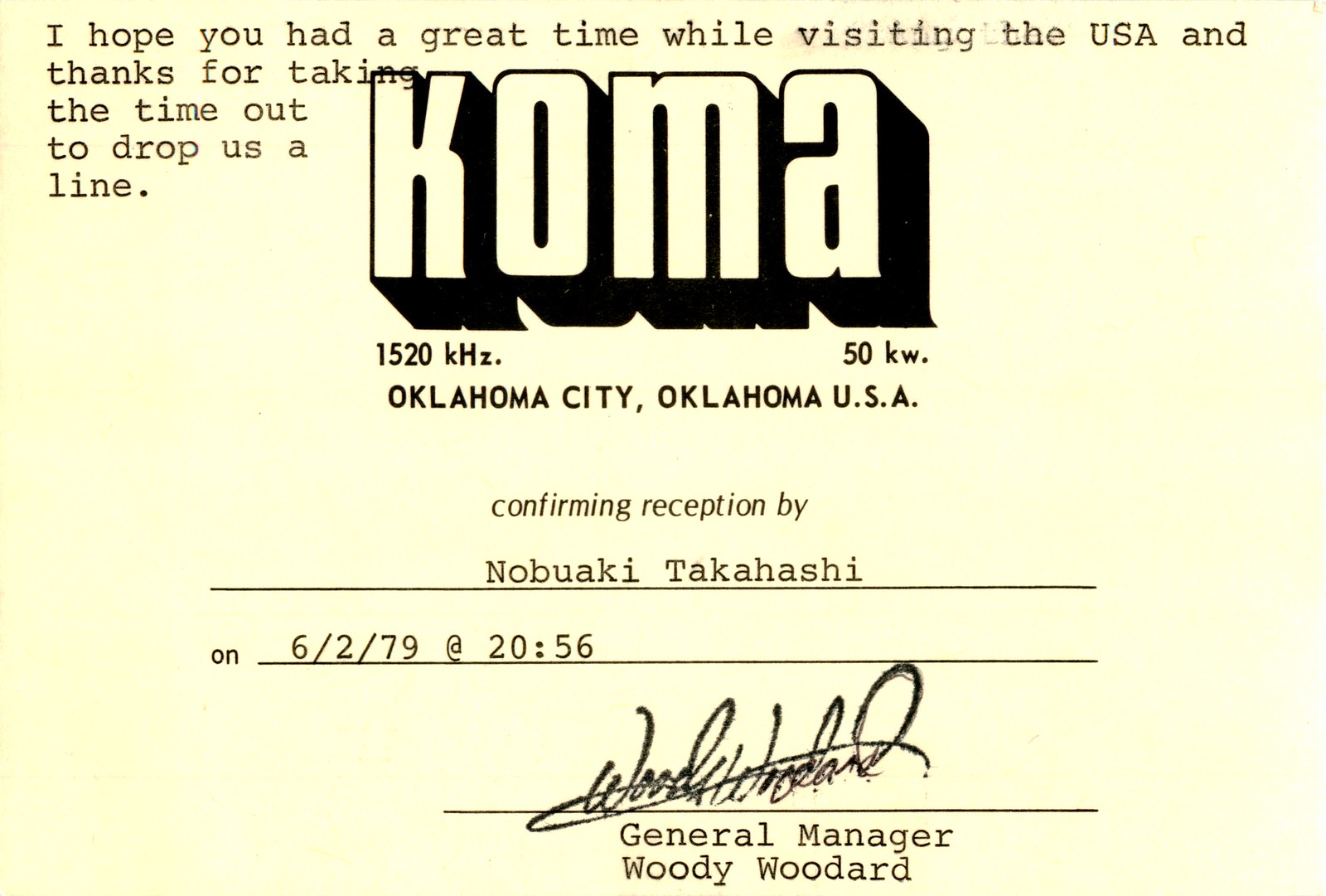The image depicts a yellow piece of paper with black text, appearing to be some sort of confirmation receipt or acknowledgment. At the top, it reads, "I hope you had a great time while visiting the USA and thank you for taking the time out to drop us a line." Below this, in bold black text, it prominently displays the logo "KOMA," followed by details indicating a radio station: "1520 kilohertz, 50 kilowatts, Oklahoma City, Oklahoma, USA." Further down, it states, "Confirming reception by Nobuaki Takahashi," with the date "6-2-79" and the time "2056" in military format. The document is signed in cursive by the general manager, Woody Woodward, with his title listed below the signature.